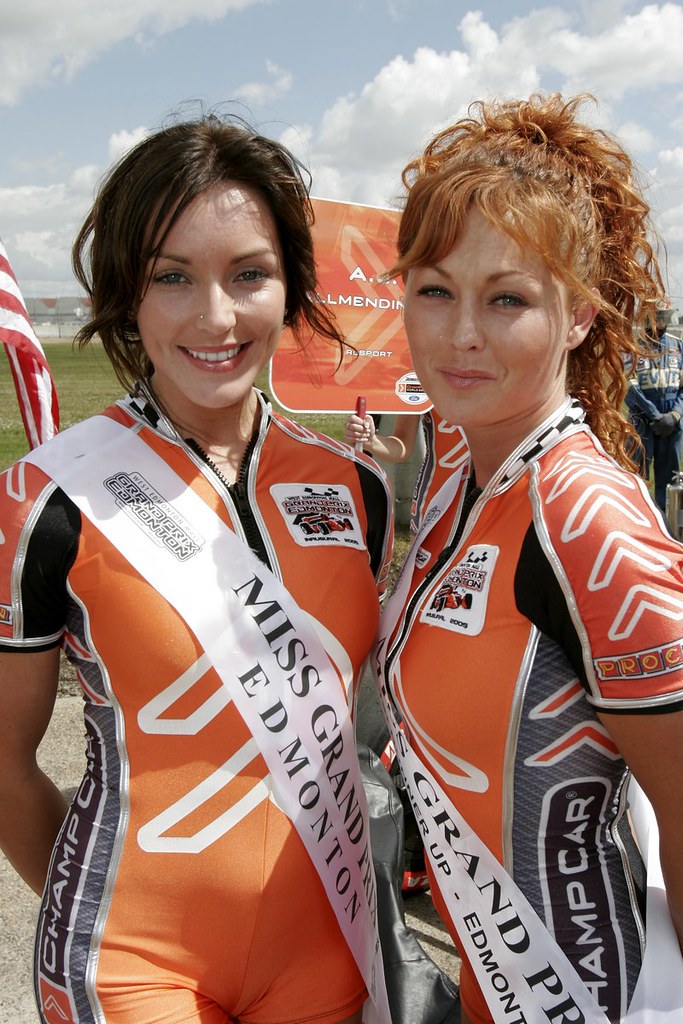The photograph features two female models prominently posed in front of a racing team backdrop, on a cloudy, overcast day with hints of green grass and an American flag in the background. Both women, wearing matching tight-fitting athletic racing bodysuits in orange with black and white detailing, stand side by side smiling and looking directly at the camera. Each has a white sash draped over her right shoulder that identifies them as participants in a Miss Grand event associated with Edmonton. The model on the left has short black hair, while the model on the right sports shoulder-length, curly red hair. Behind them, additional figures in racing uniforms and an orange sign can be seen, contributing to the dynamic and energetic atmosphere of the scene.